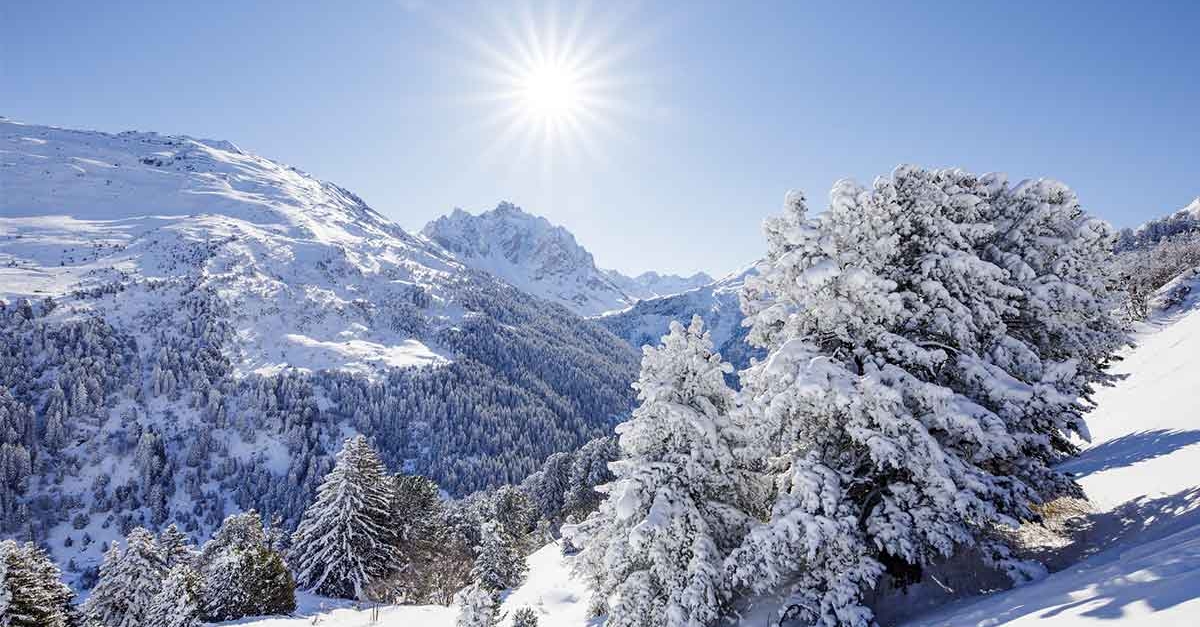An absolutely stunning nature photograph captures a snow-covered Nordic-like landscape, possibly situated in North America, such as Canada or Montana. The scene is dominated by towering, snow-capped mountains that stretch across the horizon on the left and right, meeting a perfectly clear, vibrant blue sky devoid of clouds. The sun, bright and white, is positioned slightly to the left of center and casts radiant beams that illuminate the landscape, creating long shadows behind the trees and enhancing the crispness of the freshly fallen snow.

The foreground is adorned with numerous evergreen trees, predominantly pines and spruces, their boughs heavily laden with fresh snow that droops under its weight. These snow-covered trees populate both the right side of the image and the central area, contributing to the serene and pristine atmosphere. Additionally, a prominent evergreen bush stands right in front, its dense foliage blanketed by the snowfall.

Furthermore, the rocky, gray surfaces of the mountains are partially visible through the snow, adding texture and contrast to the scene. The tree line ascends about a third of the way up the mountains before giving way to pure, untouched snow higher up. Overall, the entire composition exudes tranquility and natural beauty, highlighted by the absence of text, allowing the viewer to fully immerse in the snowy, sunlit wonderland.